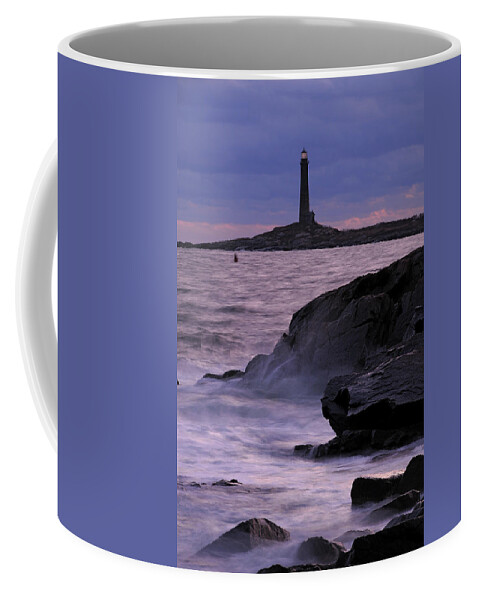The image depicts a navy blue coffee cup with a white handle and interior. The cup features a detailed seascape with a tall, slim lighthouse standing on a rocky island. The lighthouse has a yellow light and is framed by a dusky blue sky, matching the cup's exterior. In the scene, choppy waves with whitecaps crash onto large black rocks in the foreground. Smaller rocks and a buoy bobbing in the water add to the turbulent ocean setting. The surrounding mist from the splashing waves enhances the atmosphere of a stormy, challenging place for sailors.